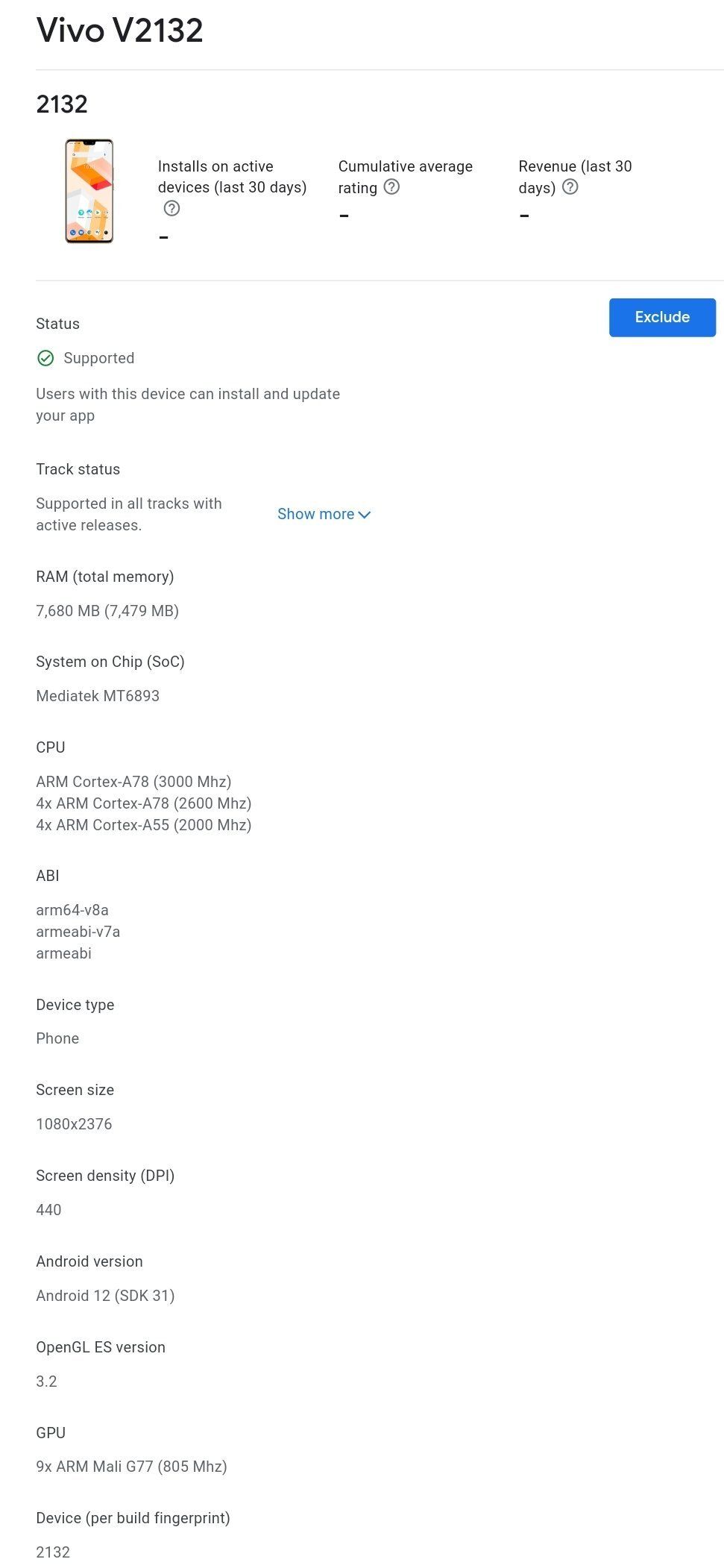The screenshot depicts a section of a cell phone screen. In the upper left corner, the text "V2132" is prominently displayed. Below this, the same text "V2132" is reiterated, accompanied by a graphic of a phone and a note indicating that the app has been "installed on an active device in the last 30 days." To the right, there is a field that displays the average ratings for the app. This layout is repeated multiple times below, making for a redundant series of entries, each stating "V2132," alongside the phone graphic and the 30-day install notification.